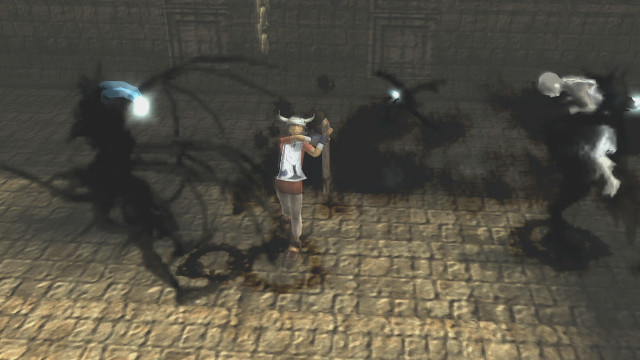In this screenshot from a video game, the scene unfolds on a cobblestone street or road, surrounded by stone buildings with wooden doorways. At the center of the image stands a character, possibly female, donned in a metal helmet with Viking-like horns. She wears a white vest over an orangey-red shirt, white pants, and shoes, and wields a long, light-brown weapon—a sword or an axe. The graphics, though not the best, show shadowy, smoky shapes all around. To the right, a creepy, glowing, white figure with a bald head hovers, wrapped in shadows, suggesting a ghostly presence. Other shadowy creatures also appear in the scene—one with a blue head and white light in its smoky body, another seemingly carrying a human soul-like figure, white and transparent. The ground features strange markings on the cobblestones, adding to the eerie and chaotic atmosphere of the game’s castle-like dungeon setting.